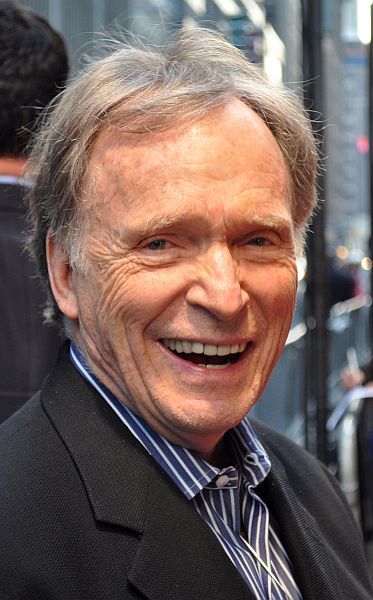This is a detailed color close-up photographic portrait of Dick Cavett, the renowned television personality and long-time interviewer from late-night television. The photo captures him from the shoulders up, with a clear view of his thinning gray hair and light blue eyes. Smile lines and wrinkles mark his face and forehead, adding character to his warm expression. He is dressed in a black suit jacket over a blue-and-white striped collared shirt, with a white button clearly visible. Cavett is smiling at the camera, his teeth prominently showing. The outdoor setting reveals a blurred daytime cityscape in the background, highlighted by the reflective windows of an office building. Directly behind Cavett, to the left, stands a man with short dark hair, wearing a gray suit jacket over a blue shirt, facing away from the camera. The black frame of one of the windows can be seen to the upper right of Cavett, contributing to the urban ambiance of the scene.